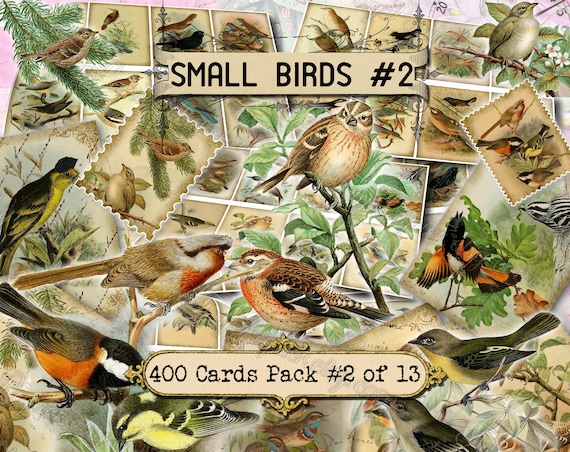The image is a detailed, chaotic collage of colorful bird illustrations arranged to resemble postage stamps, clearly put together digitally, likely in Photoshop. Titled "Small Birds Number 2" and labeled as part of a "400 Cards Pack Number 2 of 13," the composition features a mosaic of variously shaped and sized stamps showcasing an array of old-school illustrated birds. These birds have distinctive colorations, including yellow, grey, and orange bellies, and some are depicted perched on branches. The overall design simulates the look of a vintage stamp collection, complete with simulated paper texture and stamp-like ridged edges, giving a preview of the collectible cards within the pack.